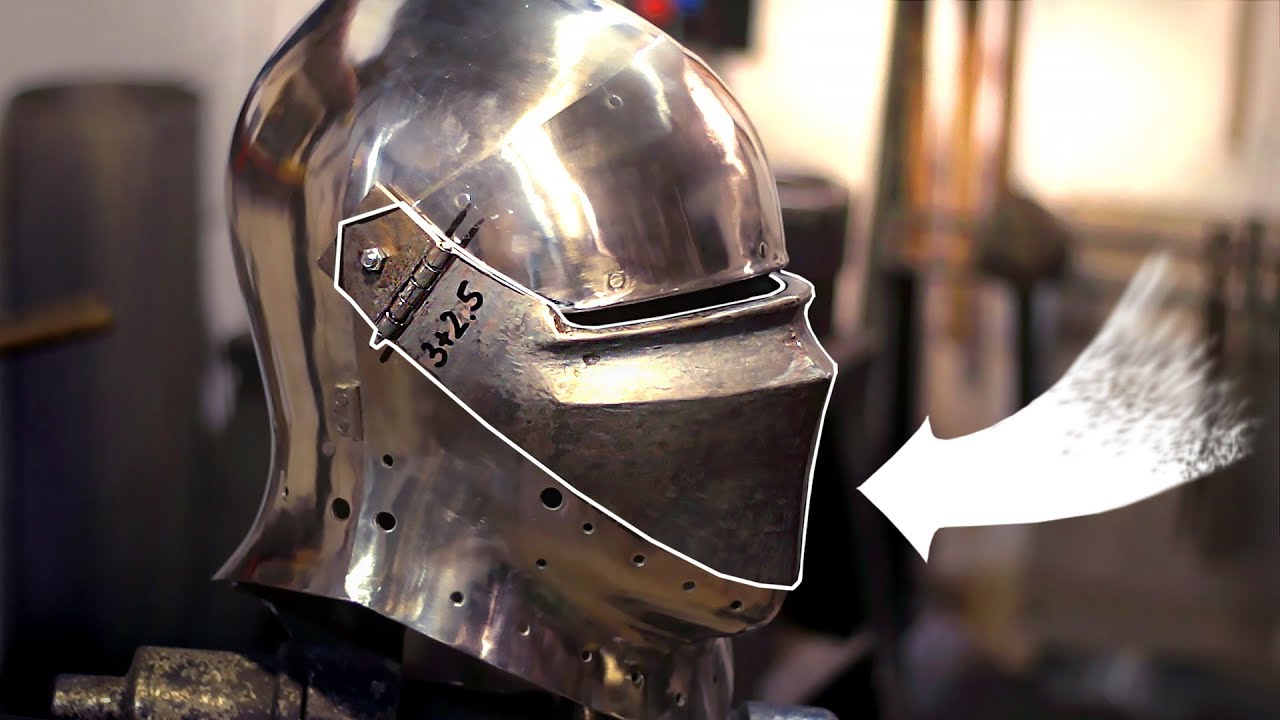This enchanting image captures the meticulously maintained right profile of a knight's helmet, gleaming under the light. The high polish on the helmet leaves it uncertain whether it is a contemporary creation, an exquisite reproduction, or an immaculately preserved artifact from the past. The focal point of the image is the helmet's intricately crafted mouthpiece, accentuated by a delicate white stroke outlining its form. A white arrow prominently points towards the mouthpiece, drawing attention to its intricate details. Curiously, along the side of the mouthpiece, the inscription "3+2=5" can be seen, adding an element of mathematical intrigue to this historical piece of armor.